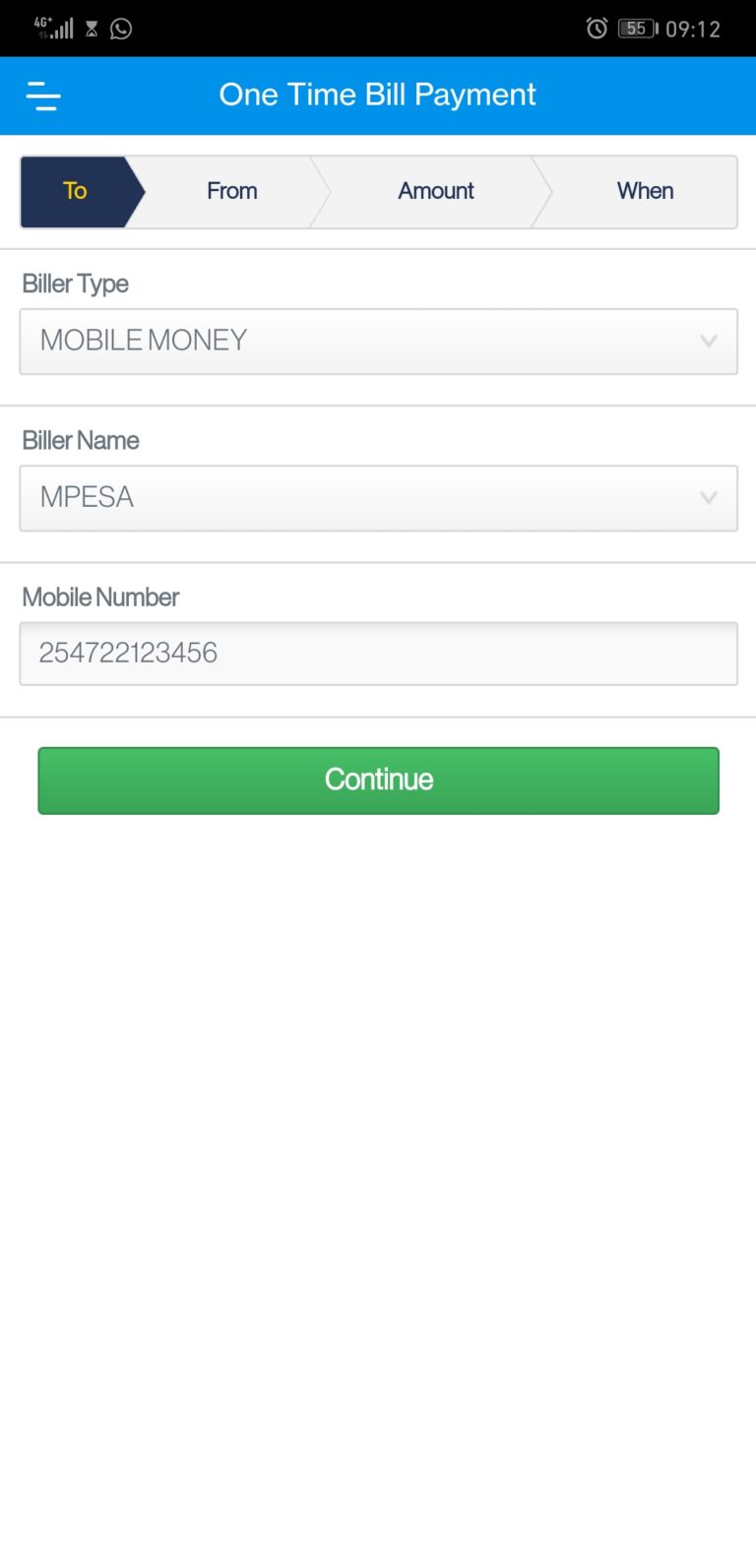An image displays a mobile phone screen showing an online bill payment interface. At the top, a blue header prominently features the text "One Time Bill Payment" in white letters. Below this header, there are four selectable options arranged horizontally: "To," "From," "Amount," and "When." The "To" option is currently selected and is highlighted with a navy blue background and yellow text, while the remaining options have a grey background with black text. 

Following these options, a series of fields and selections are visible. The first field is labeled "Biller Type" and is filled in with "MOBILE MONEY" in all capital letters. Next, the field labeled "Biller Name" contains "M-P-E-S-A," also in all caps. Further down, there is a field for "Mobile Number," which displays the number "254722123456." 

Directly below these fields is a green button with the word "Continue" in white letters, outlined by a black border. The top of the screen shows common mobile phone status indicators, including a black border, the current time, an alarm clock icon, the WhatsApp icon, signal strength, and other standard features.